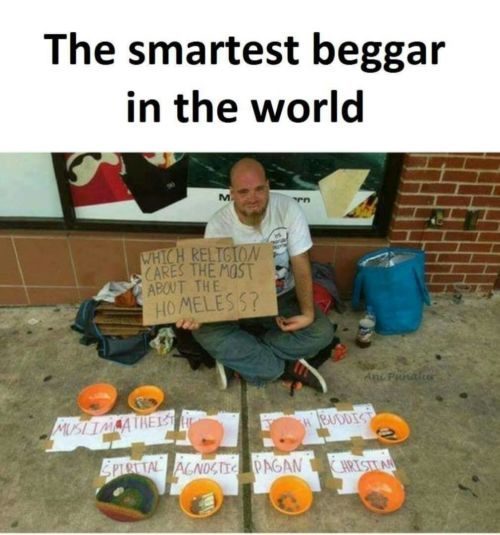This image depicts a bald, bearded homeless man sitting cross-legged on a dirty city street sidewalk, possibly in front of a fast-food restaurant. Above him, the caption "The Smartest Beggar in the World" is displayed in black text against a white background. The man is casually dressed in a white t-shirt with some lettering and blue jeans, and he has scattered possessions including a blue bag to his right and other belongings to his left, along with a bottle that appears to be Pepsi. 

He is holding a cardboard sign that reads, "Which religion cares the most about the homeless?" In front of him on the sidewalk are nine bowls, each placed on a piece of paper labeled with a different religious or belief system: Muslim, Atheist, Agnostic, Spiritual, Pagan, Buddhist, Christian, with the last two partially obscured but likely Hindu and Jewish based on the context. Each bowl contains varying amounts of currency in both coins and paper bills. The surrounding environment features dirty tiles to his left, a brick wall behind him with an indistinguishable sign, creating a stark and poignant scene that the man acknowledges with a slight smile directed at the photographer, suggesting the image was taken in a casual, non-professional manner from an overhead angle.